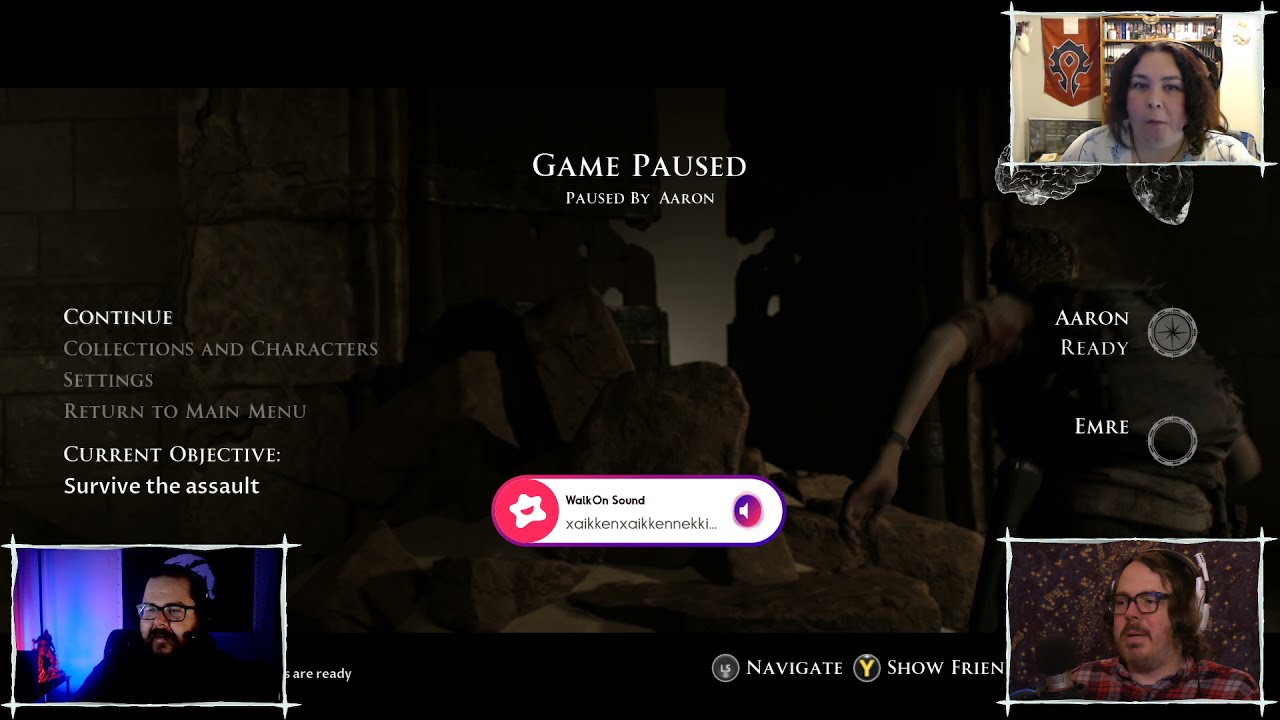The image is a detailed screenshot or pause screen from a video game, possibly captured during a Twitch stream. The background is shaded out, highlighting the menu options and player information prominently displayed on the screen. The menu on the left lists several options in white text: "Continue," "Collections and Characters," "Settings," "Return to Main Menu," and "Current Objectives," with the specific objective being "Survive the Assault." 

At the center of the screen, the words "Game Paused, paused by Aaron" are visibly written. On the right side, two circles indicate player statuses: "Aaron Ready" (highlighted with an icon) and "Emery." Below these, there are options for "Navigation" and "Show Friends."

The screen also displays small, framed webcam feeds of three players in the corners: 
- The top right shows a red-haired woman with a slight smile or eating, set against a white wall with a bookshelf and a medieval-style red flag.
- The bottom right showcases a man in an orange plaid shirt, big glasses, a mustache, and white headphones, appearing to be speaking.
- The bottom left features another man with glasses and a large mustache, sitting in a dimly lit room with purplish-pink lighting.

Additionally, a red pop-up in the center reads "Walk On Sound" with a series of random letters, and a hot pink circle with a smiling star can be seen on the left part of the screen.